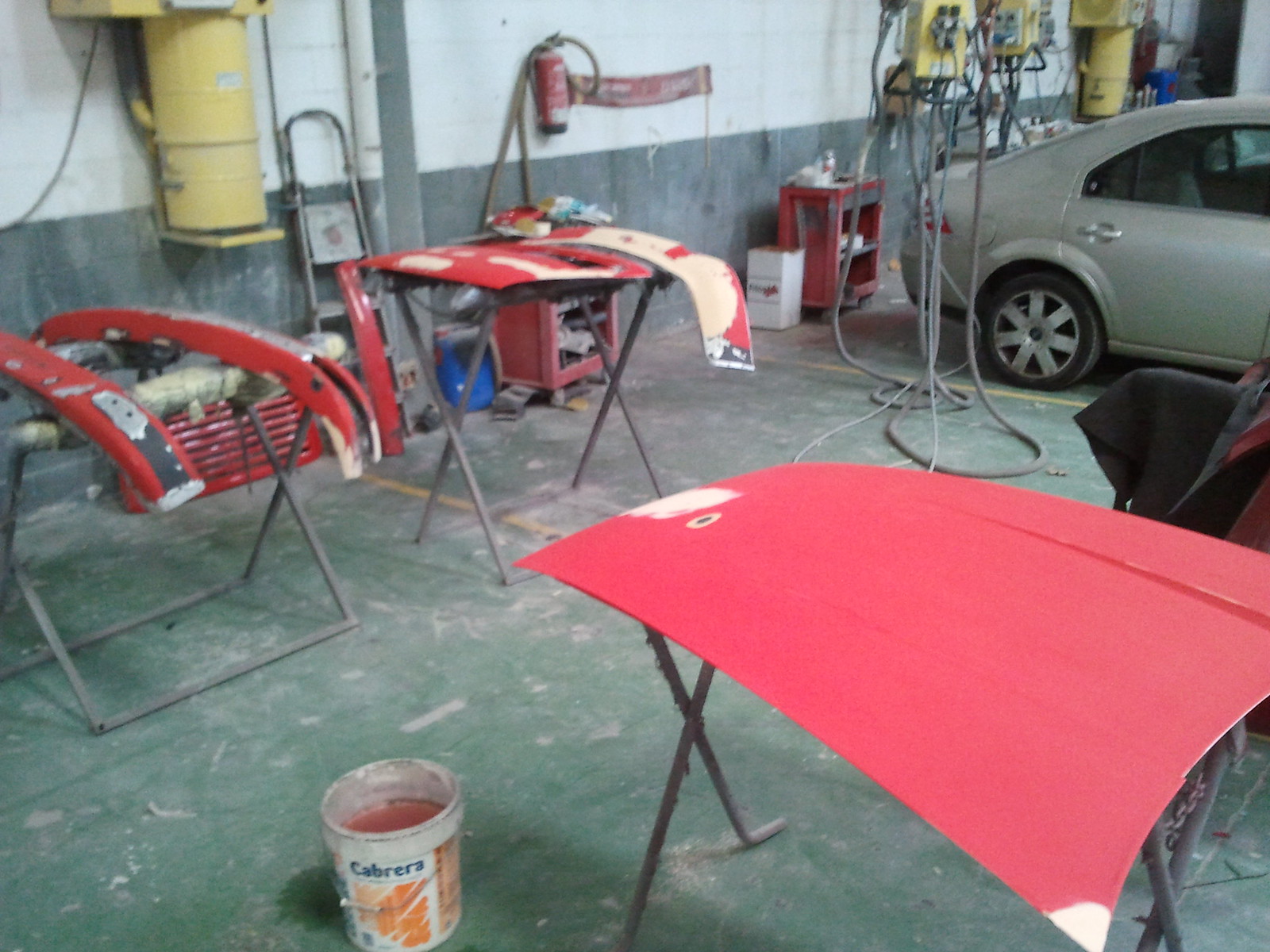The photograph depicts an industrial automotive garage with a cluttered yet organized workspace. In the upper right corner, a gray car is partially visible, parked against the white cement walls with a black lower section. The garage floor is dirty cement, littered with various tools and equipment. Several car body parts, including a red hood and bumpers, are elevated on metal stands, indicating ongoing work. A white bucket with 'Cabrera' written in blue letters and orange accents, filled with strange grayish-red liquid, is positioned near the front left of the image. Yellow machinery, likely a car lift, and a red cabinet about two and a half feet high containing tools are also present. Additionally, a red fire extinguisher is mounted on the wall, and a stepladder leans against it. The scene is accentuated by the industrial feel of the space, marked by pipes and mechanic equipment on the walls.